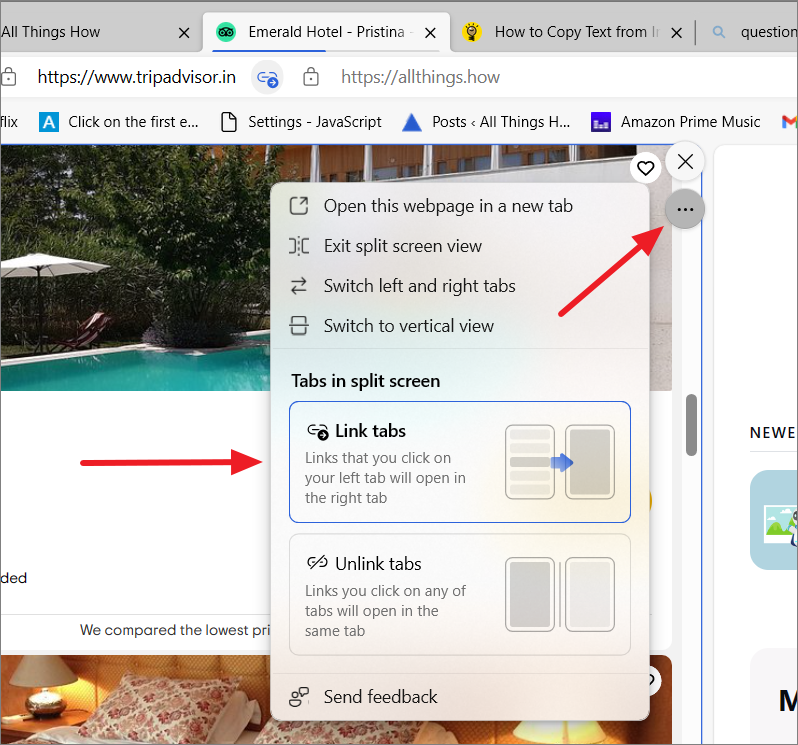A detailed screenshot of a computer displaying the website "All Things How" is shown. A pop-up menu overlays the main content, offering options like "Open this web page in a new tab," "Exit split screen view," "Switch left and right tabs," and "Switch vertical view." Below these options, there are sections labeled "Tabs in split screen," which features linked and unlinked tabs. 

The first tab, highlighted with a blue border, contains two subsections:
1. **Linked Tabs** - Links clicked in the left tab will open in the right tab.
2. **Unlinked Tabs** - Links clicked will open in the same tab.

Behind this menu, the content relates to hotel information, featuring images of a swimming pool and what appears to be a hotel room. Moreover, the browser's top border contains several tabs, including "Click on the first E ellipses," "Settings," "JavaScript," "Posts," "All Things Hotel," "Amazon Prime Music," and "Google Gmail." The context suggests that the website being viewed is part of Trip Advisor, geared towards hotel-related content.